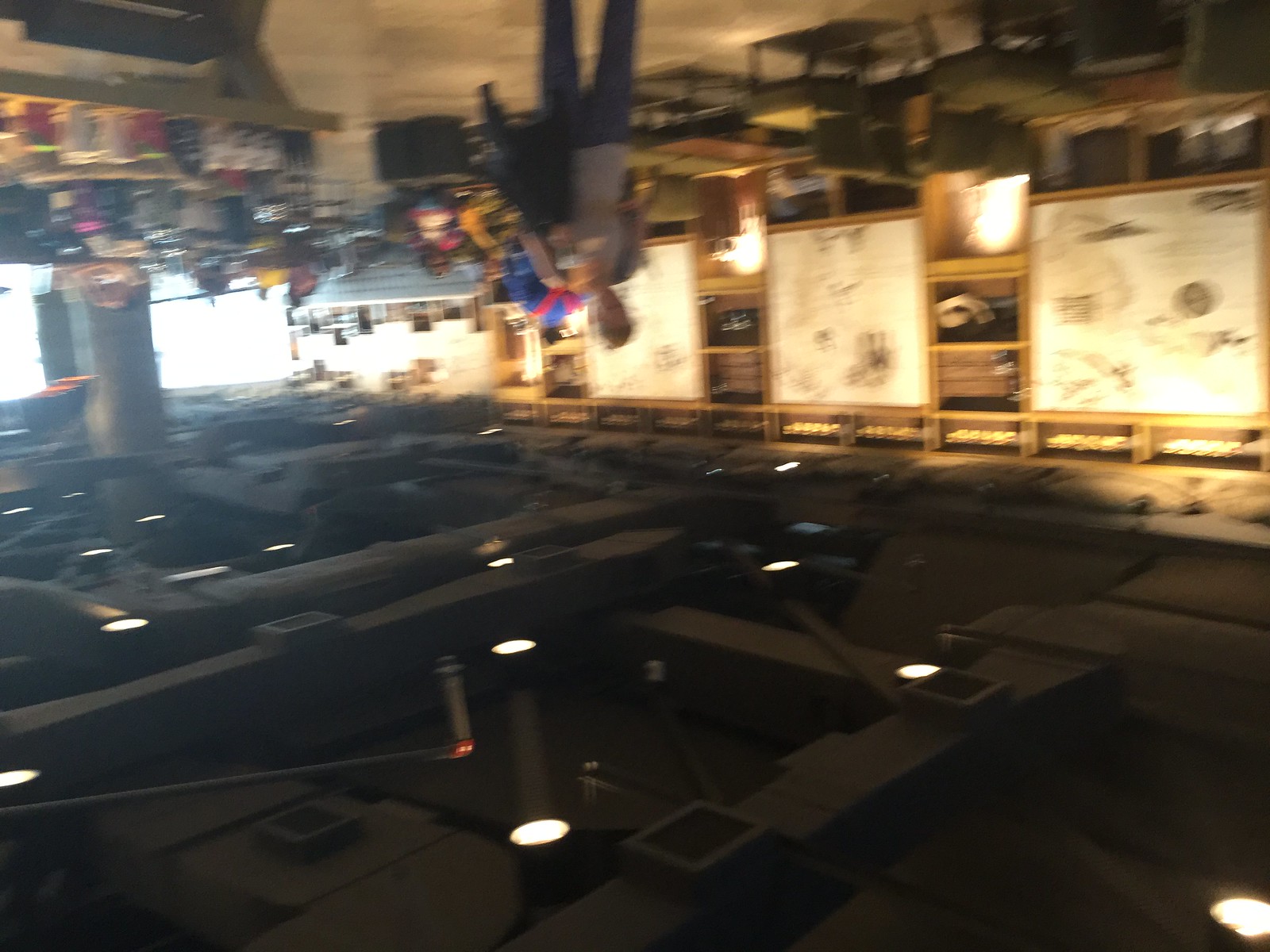This photograph, which is both blurry and upside down, captures the interior of an industrial-style building, possibly a restaurant or canteen. The ceiling, which in the rotated image appears at the bottom, showcases an exposed HVAC system painted dark, almost black, with circular black lights that illuminate the blurry figures below. Central to the image is a male figure in a gray shirt and blue jeans, facing the viewer, though his features are indistinct due to the blurriness. Surrounding him are other vague human forms, potentially people or objects. In what would be the lower right-hand corner if the image were right-side up, there appears to be a sales counter with drink cups lined along its base, suggesting the availability of snacks and beverages. The cream-colored floor and walls, adorned with some design or wallpaper, and the presence of tables and chairs, indicate a bustling indoor environment. In the top left corner, there seems to be a buffet bar or similar setup. Brightly colored coffee mugs and gold-hued elements are scattered throughout the mid-ground, adding to the detailed complexity of the scene.